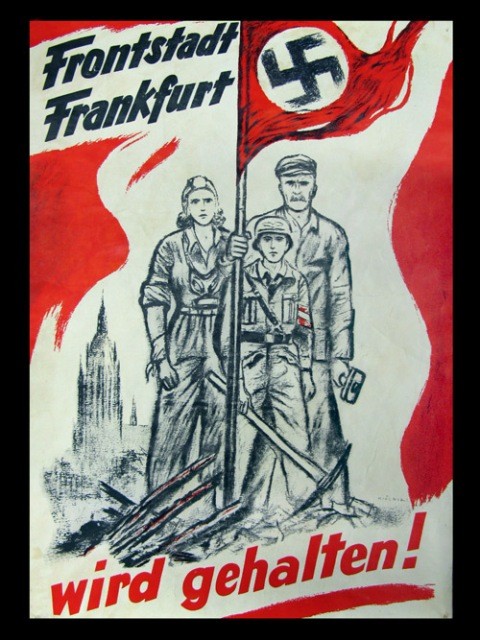This detailed, hand-drawn illustration, reminiscent of 1940s German propaganda, depicts three central figures: an older man, a young woman, and a youth, arranged around a vividly rendered Nazi flag. The flag features the prominent swastika symbol within a white circle against a red background. The man, distinguished by his mustache and cap, holds the flagpole and a hammer, while the youth, attired in a soldier’s uniform with a Nazi armband on his left arm, grips a pickaxe. The young woman, positioned to the left of the man, wears a jumpsuit, collectively suggesting a scene of wartime unity and resilience. The background faintly reveals a building amidst turmoil, accentuated by red swooshes that symbolically flow around the figures, adding to the image's dramatic impact. Above and below, the text reads "FRONTSTADT FRANKFURT" and "WIRD GEHALTEN!" in bold black and red letters, respectively, reinforcing the propagandistic message.